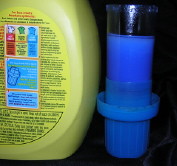In this photograph with a plumbing theme, which is set against a completely black background, we observe a symmetrical and perfectly square frame. On the left side, there is a bright yellow gallon jug resembling a laundry detergent container. Its back shows an even brighter yellow sticker detailing instructions for use, accompanied by multiple images in the center and text on the right bottom and left-hand side. 

On the right side of the image, near the jug's height, there's a blue object, which appears to be a cap associated with the jug. This cap, akin to those used for measuring laundry detergent, features a distinctive structure—a cup-like bottom with a pillar rising up, possibly to hold more liquid. This blue cap not only serves practical utility but also gives the impression of containing some blue liquid, reinforcing its functional appearance in the context of detergent storage and measurement.